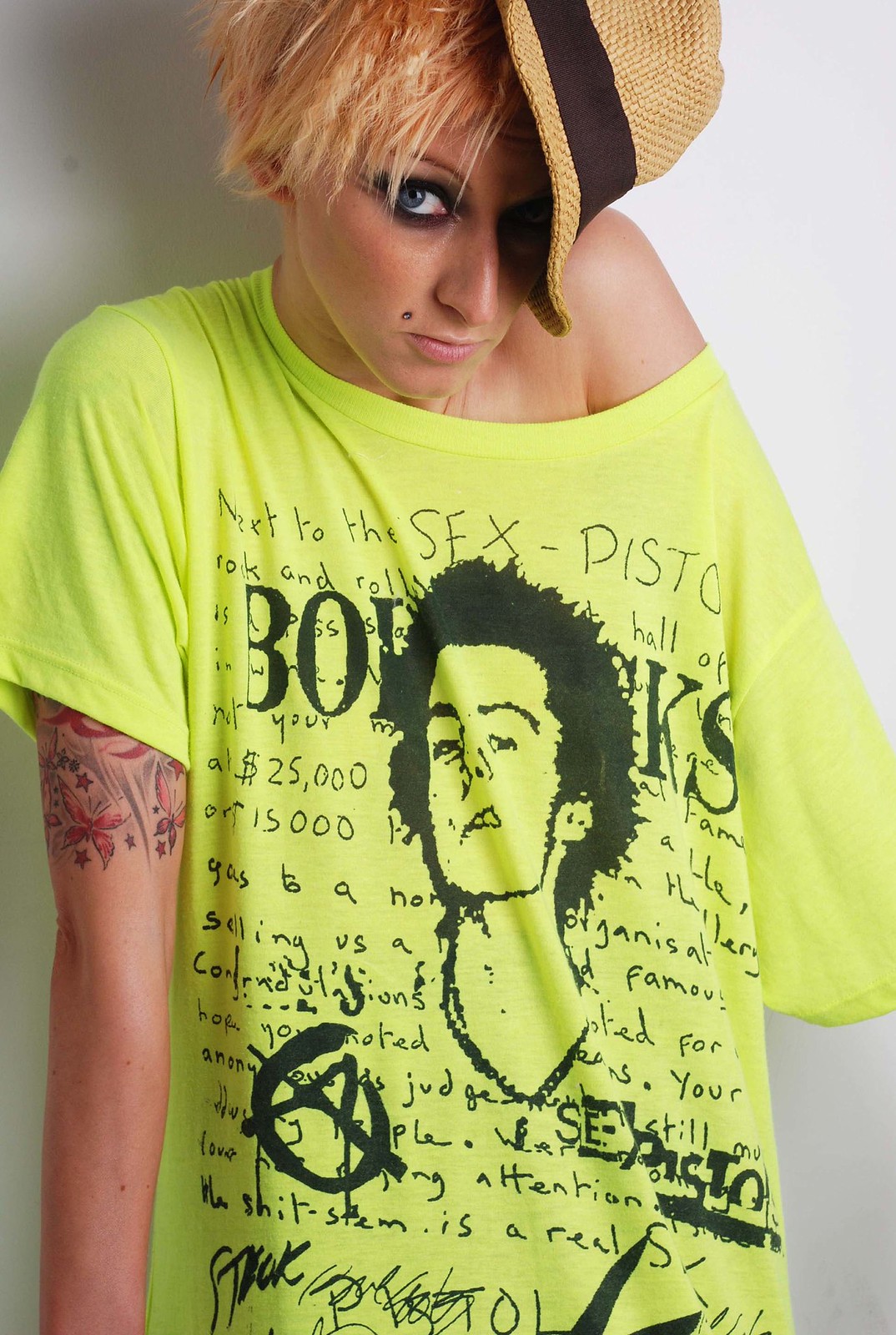In this image, we see a woman with very short, choppy hair that resembles straw, a mix of blonde, brown, and yellow hues. A straw hat sits sideways on her head, partly covering the left side of her face, which is cast in shadow. She has heavy black eyeliner and a painted-on mole just above her right lip. Her expression is serious as she looks straight at the camera.

The woman is wearing a bright yellow t-shirt adorned with various graphics and text. The t-shirt features a prominent drawing of a man's head with black hair, displaying a sneering expression with exposed teeth. The text around the graphic includes elements such as "Sex Pistols" near the top and "piston" scribbled across and around the image. There are also handwritten notes and scribblings on the shirt, including a crossed-out "A" on the bottom left part of the graphic. The right sleeve of the t-shirt is pulled down, revealing her shoulder, while just below the left short sleeve, we can glimpse a colorful tattoo featuring red and grey butterflies and stars.

Overall, the woman's striking appearance is accentuated by her intense eye makeup, short vibrant hair, and the distinct graphics on her yellow t-shirt, creating a captivating and edgy look.